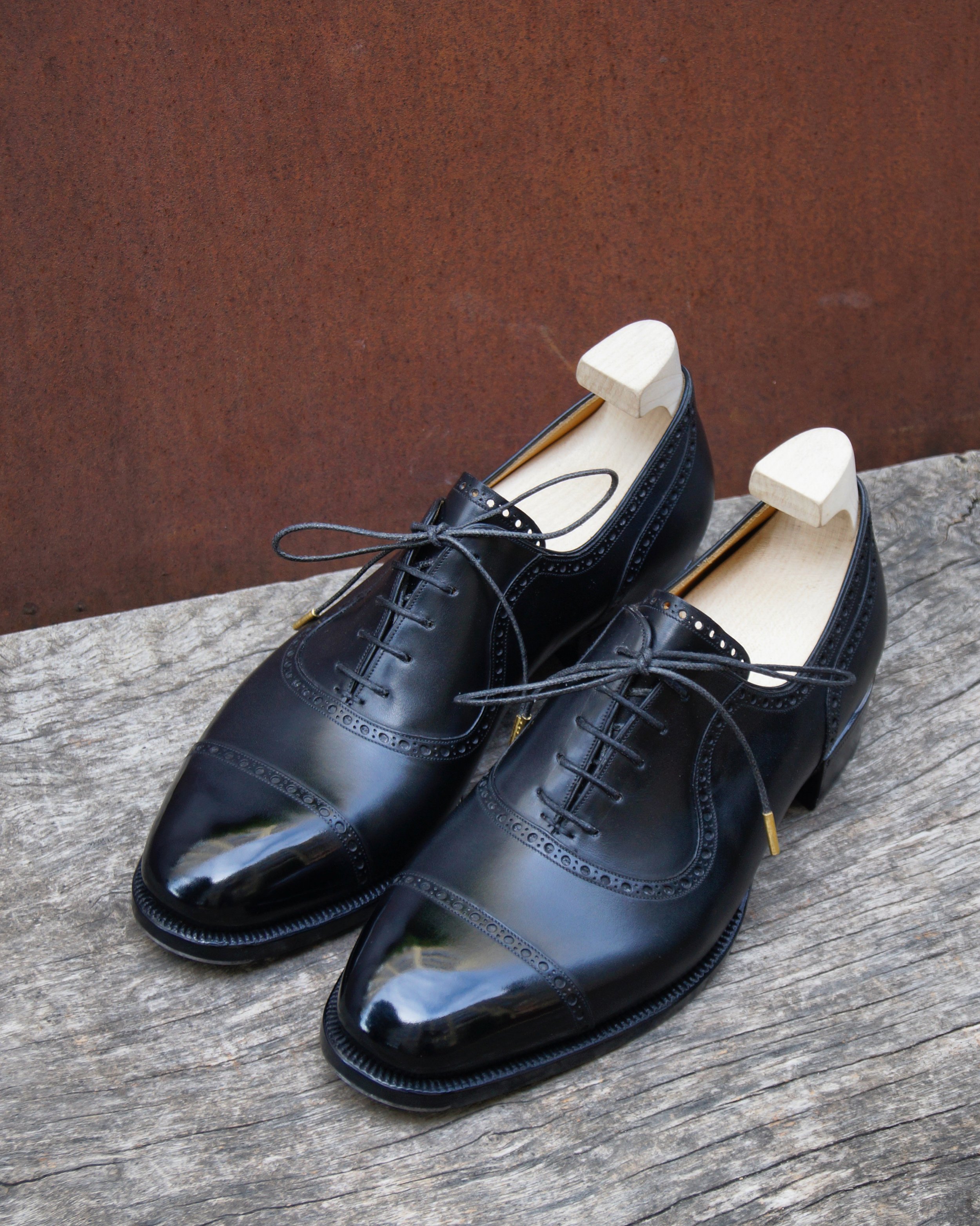This image captures a pair of meticulously detailed black leather dress shoes, characterized by their striking contrast between glossy toe caps and matte finish elsewhere. The shoes are each supported with a white wooden shoe tree featuring a handle for easy removal, showcasing shoe store presentation quality. The black round laces, adorned with small golden aglets, complement the elegant look, while decorative stitching embellishes the toe caps. The shoes rest atop a weathered, rustic wooden platform with visible cracks and varying shades of gray, giving it a rugged, outdoor picnic-table feel. Behind the shoes, a copper-brown, rusty metal sheet stands as the backdrop, featuring numerous rust spots that contribute to the vintage and handcrafted atmosphere conveyed by the scene.